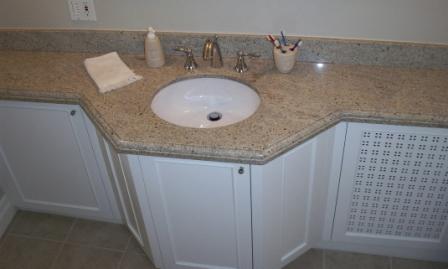This photograph captures a detailed view of a stylishly arranged bathroom vanity. The centerpiece is a white, oval-shaped basin featuring a stopper plug that can be adjusted to retain or release water. Surrounding the basin is a sophisticated rose-colored stone countertop, which complements the basin's simplicity. Just behind the basin, you can observe modern, brushed-metal fixtures that consist of separate taps for hot and cold water, along with a centrally positioned spout extending from the bench.

To the right of the basin, there is a ceramic pot with a lid, punctuated by four holes, each holding a plastic toothbrush. The toothbrushes vary in color, including blue, red, and clear. On the left side of the basin, a pale pink plastic soap dispenser with a white pump stands ready for use, accompanied by a neatly folded white hand towel positioned next to it. The vanity unit itself is finished with clean, white cupboard fronts, adding to the bathroom's overall sleek and organized appearance.